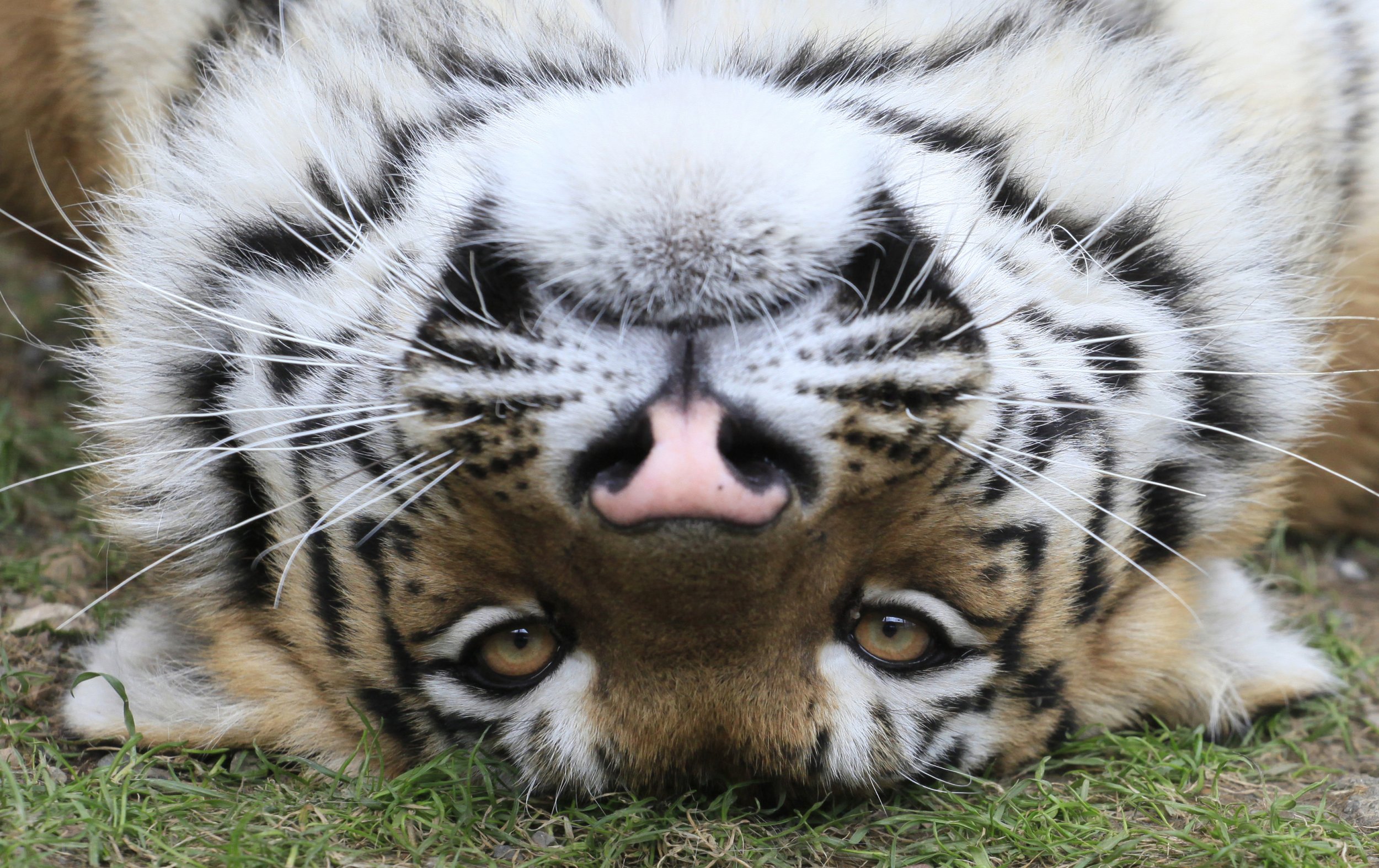This image features an intimate, close-up view of a tiger lying on its back amidst grass, with a focus entirely on its face and some upper neck and shoulder areas. The tiger's head dominates the frame, with its striking yellowish-amber eyes staring directly at the camera, conveying a calm and relaxed demeanor. The fur is detailed, showcasing the characteristic black stripes on its predominantly orange fur, which transitions to white on its chin and underbelly. You can distinctly see its pink nose with contrasting black nostrils, white whiskers fanning out from around its mouth, and the orange fur extending to its ears that have white tips. The bottom of the image displays hints of grass, further emphasizing the natural setting and the tiger's reclined position. Overall, the photograph captures the intricate details of the tiger's face up close, presenting a serene and peaceful moment in its natural habitat.